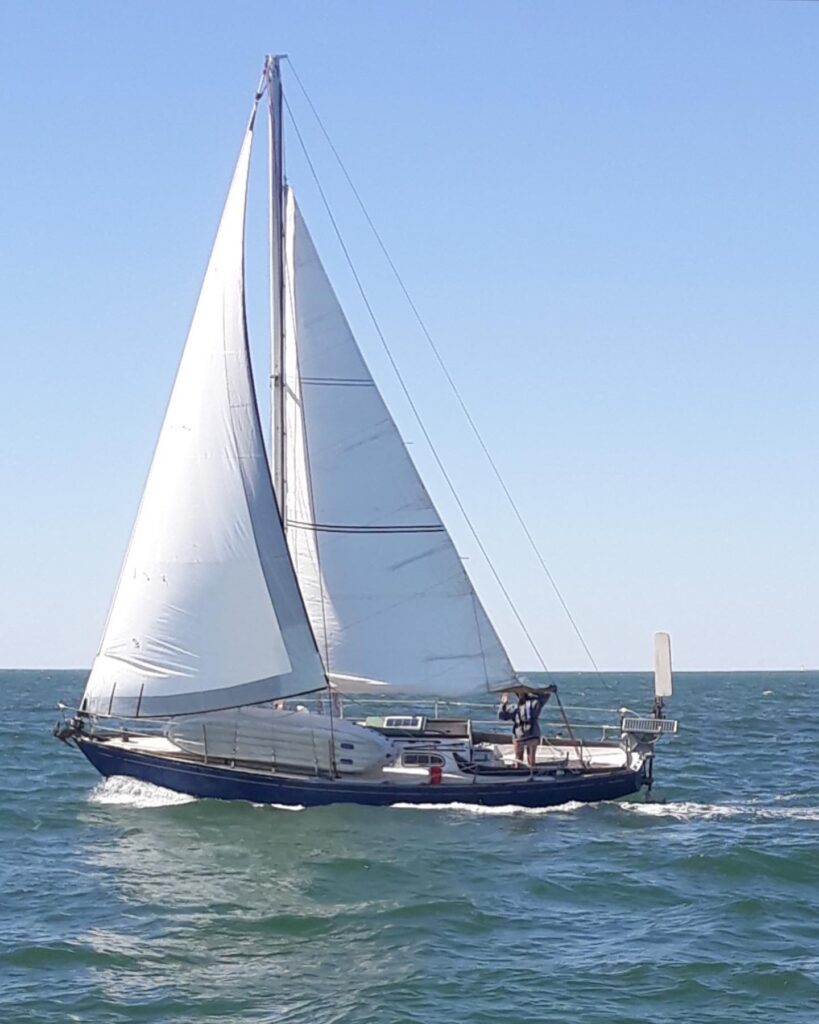This is a vertical, rectangular photograph capturing a large sailboat navigating blue waters adorned with gentle wave breaks. The background showcases a clear, azure sky above an expansive body of water with no visible horizon, emphasizing the open seas. The sailboat itself is predominantly blue on the hull with a contrasting white deck. Above the deck, two towering, white sails are anchored by a silver mast, which is supported by a network of wires. A person, bundled in warm clothes indicative of a chilly atmosphere, stands near the stern, adjusting one of the sails with both arms. This individual is nearly camouflaged by their position behind the sail steering mechanism. Adding to the details, a smaller white lifeboat is securely fastened against the metal railing that encircles the boat. At the rear of the vessel, a motor is visible, likely used for maneuvering into the harbor, and a trail of foam in its wake reveals the boat’s motion from right to left.